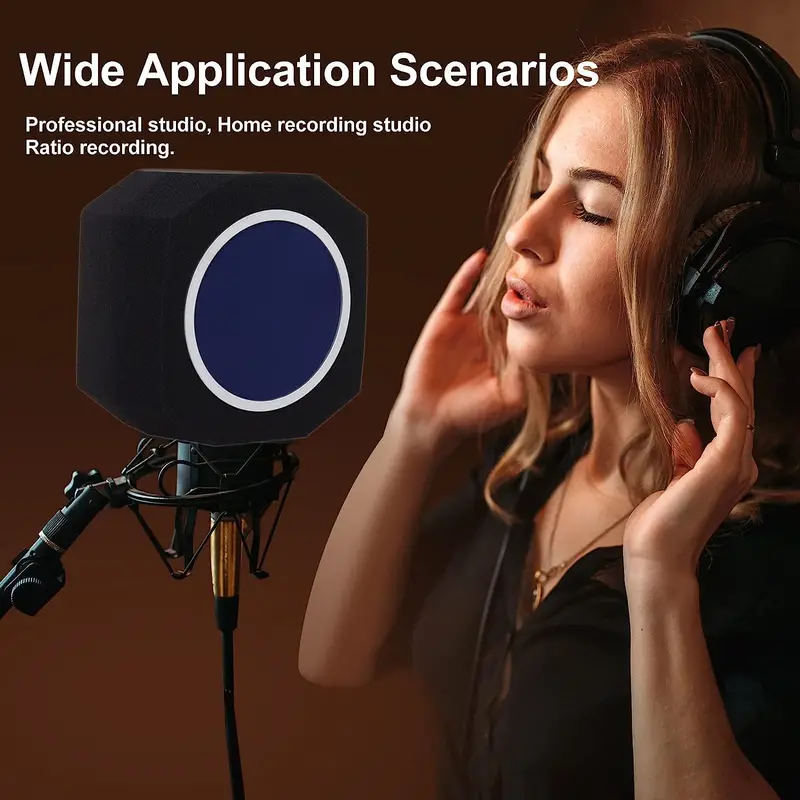This advertisement showcases a professional recording microphone, featuring a woman who bears a striking resemblance to Shakira. With honey blonde, wavy hair that's slightly past her shoulders, she exudes a composed, concentrated energy. She’s adorned in a brown shirt and wears headphones, her eyes gently closed as she sings or speaks into the microphone. Her poised hands, adorned with brown nail polish, hold the headphones firmly against her ears.

The highly detailed setup includes a microphone equipped with a shock mount extending from the left side of the frame. Surrounding the microphone is a foam isolation shield with a distinctive squarish shape, beveled at the top and bottom to encapsulate the microphone for optimal sound quality. A notable accessory, a blue pop filter with a white border, is prominently attached to the microphone.

Emphasizing versatility, the advertisement text underscores the microphone's broad application: "Wide Application Scenarios, Professional Studio, Home Recording, Studio Ratio Recording." The understated brown background further highlights the sophisticated, professional atmosphere of the recording environment.